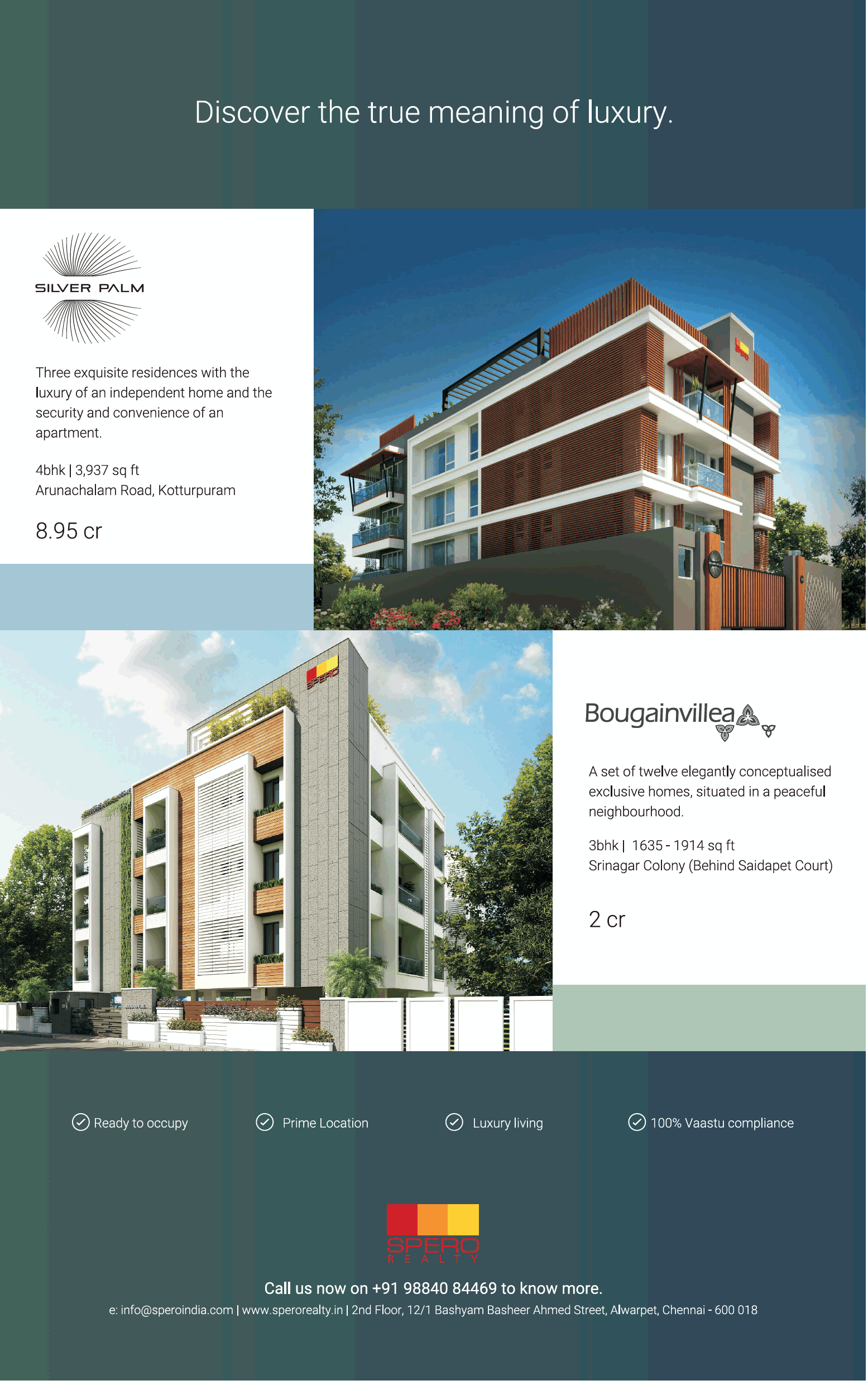The image showcases a website with a top background featuring a gradient of various shades of green. The sequence starts with a thin line of dark green, transitions into a green-teal, followed by a blue-green teal, and finally a navy blue section. Overlaying this colorful backdrop, the white text reads, "Discover the true meaning of luxury." The text is capitalized with the phrase ending in a period.

Below this section, there is a prominent white square containing text about a property called "Silver Palm." The description highlights "three exquisite residences with the luxury of an independent home and the security and convenience of an apartment," priced at 8.95 CR. Adjacent to this text, on the right side, an image of a building is displayed against a backdrop of a blue sky, dotted with a few clouds and surrounded by trees.

Further down, on the left, there is another visual of a building under a blue sky with scattered white clouds and trees flanking both sides. The text next to this image describes another property named "Bougainvillea," spelling out B-O-U-G-A-I-N-V-I-L-L-E-A, and mentions its price of 2 CR.

A sage banner appears next, followed by a section at the bottom that mirrors the initial color scheme. This segment highlights features such as "ready to occupy," "prime location," "luxury living," and "100% VAASTU compliance," with the VAASTU acronym capitalized.